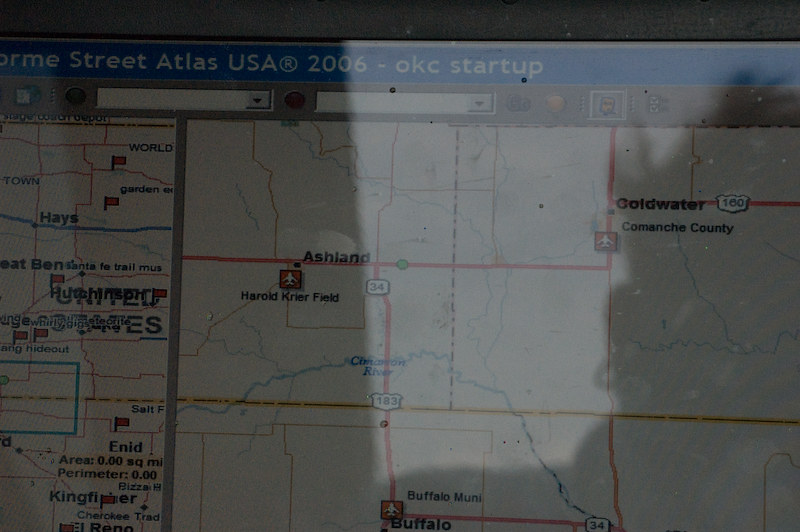This rectangular image, oriented horizontally, captures a laptop screen displaying a detailed map interface. The laptop screen prominently features the "Street Atlas USA 2006-OKC Startup" title in white text against a blue banner at the top. Beneath this, a gray banner hosts several dropdown options. The map interface shows various place names including Ashland, Harold, Cryer Field, Highway 34, and Highway 183, as well as Goldwater and Comanche County.

The image itself is taken from behind the person using the laptop, casting a noticeable shadow over the picture. The shadow allows visibility of the person’s hair, an ear adorned with an earring, part of the collar, and a fragment of the shoulder. The left side of the image is dominated by a darker shade, likely caused by the light source positioned behind the photographer.